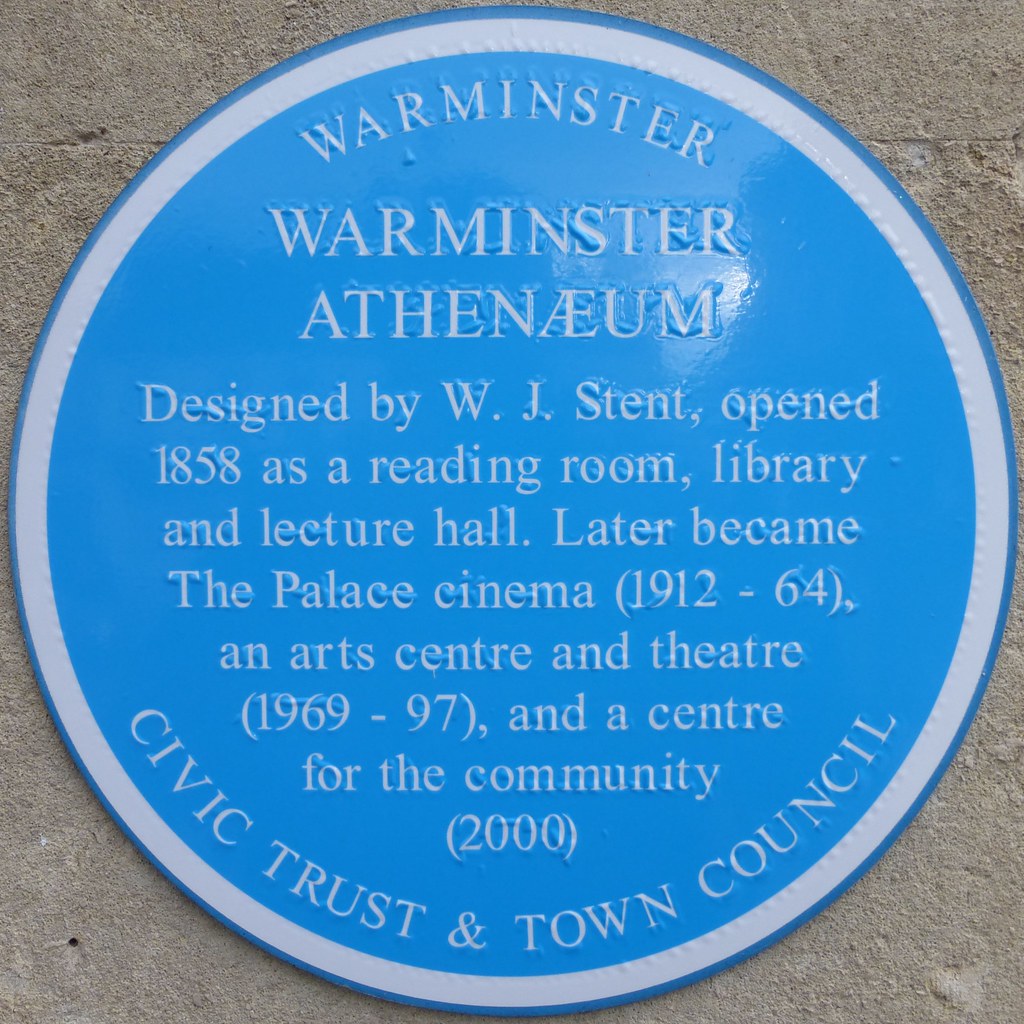The image shows a large, round blue plaque affixed to or hanging on a gray concrete wall. The plaque has a light blue center with a white border running along its circumference. In white text, it prominently reads "Warminster" at the top, followed by "Warminster Athenaeum." Further down, the text notes it was "designed by W.J. Stent, opened in 1858 as a reading room, library, and lecture hall." The plaque details its historical usage: "Later became the Palace Cinema, 1912-64, an arts center and theater, 1969-97, and a center for the community, 2000." Along the bottom curve, the text reads "Civic Trust and Town Council." The entire description and historical significance of the building are captured on this big, circular blue sign.